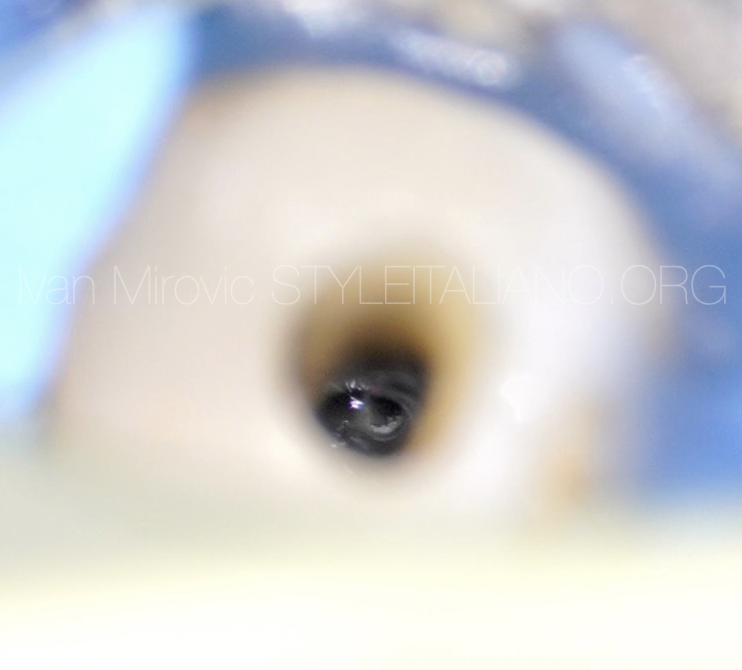The image is a square, approximately five inches in both height and width. It is exceptionally blurry, which makes identifying its contents challenging. At the very center, there is a black, rounded, spherical area with a shiny highlight accented by a touch of white. This central sphere is surrounded by a tan-colored outline, giving it depth and the impression of being nestled within a recessed space. Surrounding this, a frosted white circle covers a significant portion of the picture, reminiscent of the glaze on a donut. The upper left of the image features a brilliant, bright bluish light that transitions to darker shades of blue towards the right side. The edges of the donut-like shape exhibit hues of blues and greens, though in muted and soft tones. Across the center, from left to right, thin white lettering reads "Ivan Mirovic, styleitaliano.org." This description suggests an image that resembles a frosted donut inside a blue napkin, enhanced by a soft and blurry overlay.